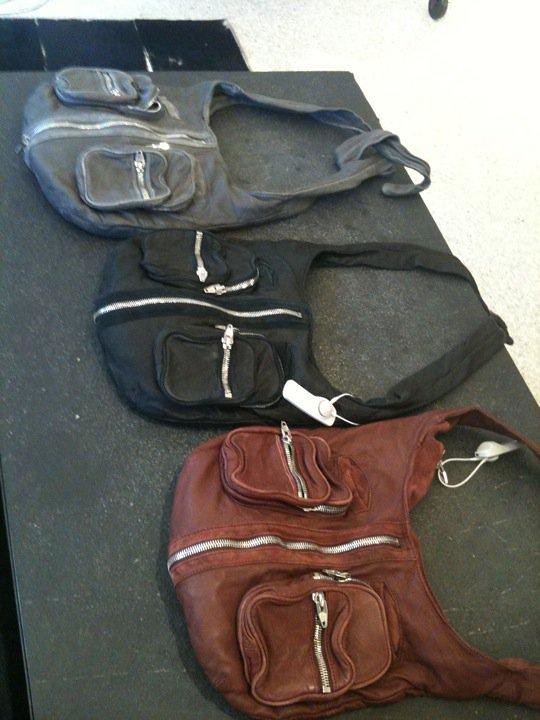This color photograph depicts three purses laid out on a table that appears to be in a low-budget store or possibly a yard sale setting. The table's gray surface contrasts with the dark green backdrop. The purses, identical in design but differing in color, are positioned from top to bottom: gray, black, and reddish-brown, with the reddish-brown being closest to the viewer. Each purse features several compartments highlighted by silver zippers, including a main zipper running down the center and two elevated square pockets with additional zippers on the left and right. The purses, possibly made from leather or nylon, seem worn and lack structure, giving them a flimsy appearance. Notably, the black and reddish-brown purses have white anti-theft tags attached, suggesting they were intended for retail but are now in a secondhand setting. The odd presence of these tags adds an element of mystery to the scenario.